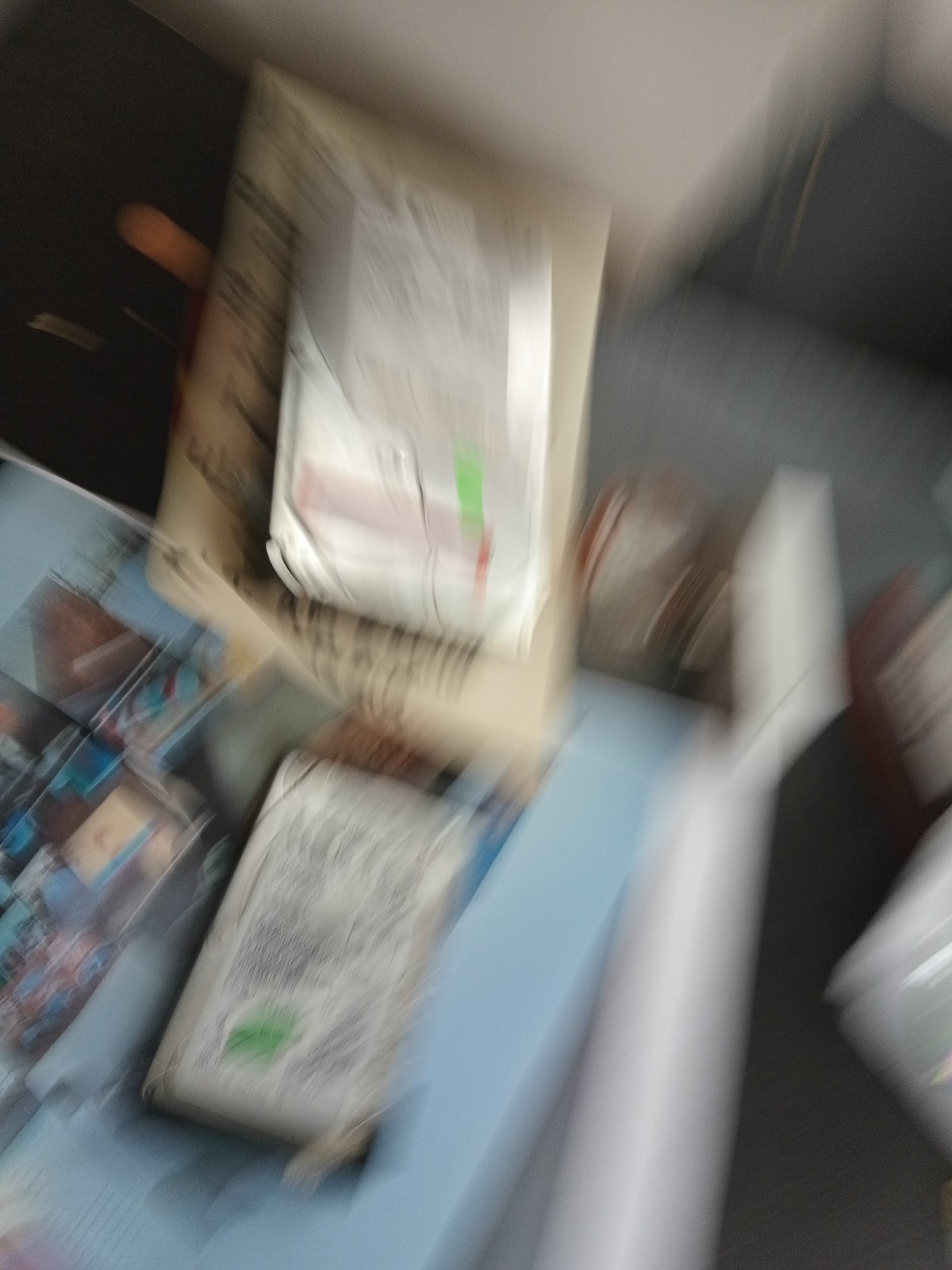This image depicts an extremely blurred scene, likely captured with the camera in motion, making it difficult to discern distinct details. At first glance, it appears to show a tabletop, possibly light blue in color, accompanied by a white chair. A grey floor can be vaguely seen beyond these objects. The scene seems to be an overhead view of a room, potentially featuring a table, a chair, and some cushions scattered on the floor. The predominant colors in the image are light blue, grey, and white. The photograph is rectangular, oriented with its longer sides vertically. However, due to the significant motion blur, the precise details and clarity of the scene remain obscured.